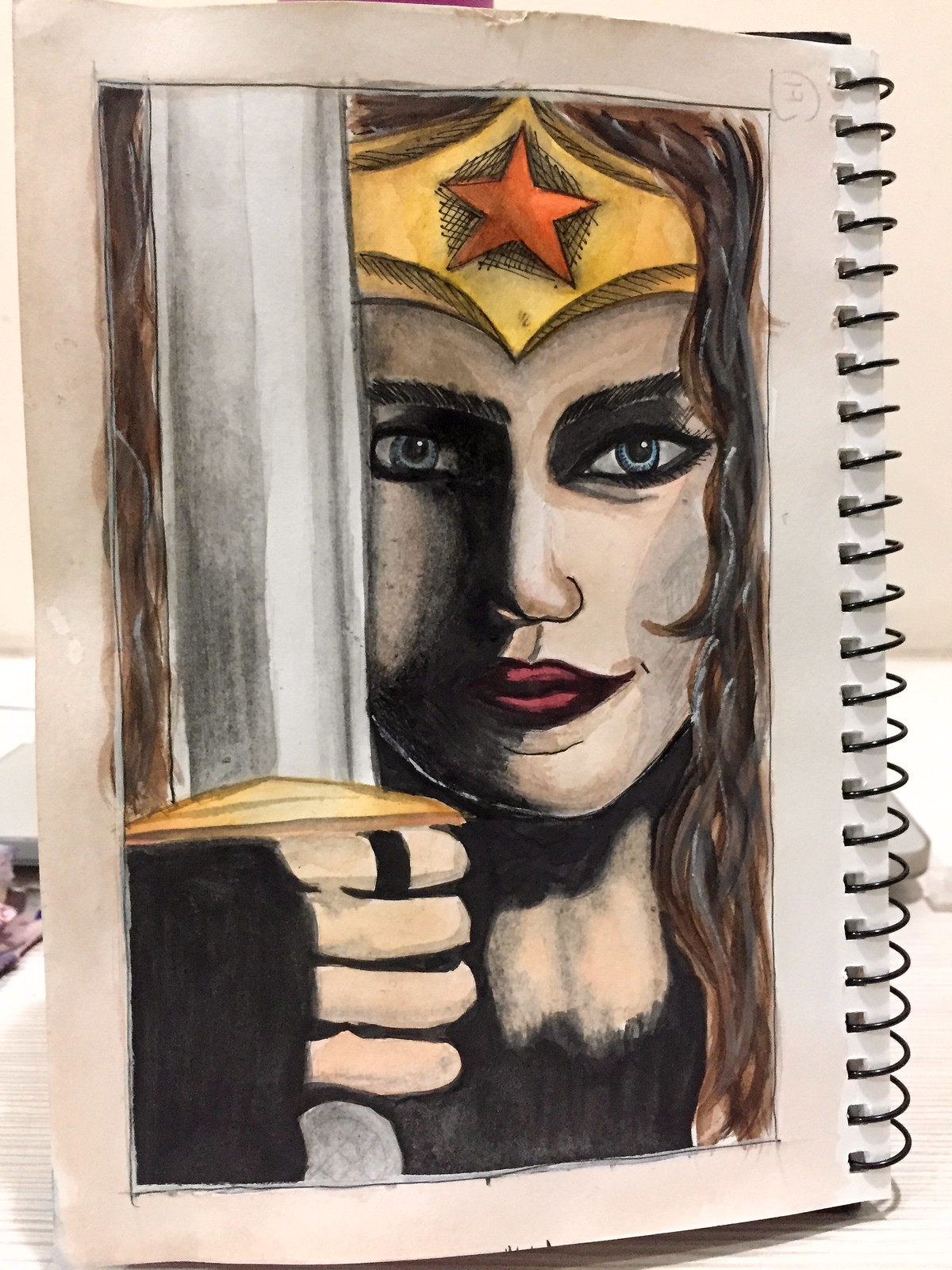This is a detailed photograph of a drawing from inside a sketchbook, with the spiral binding visible along the far right side of the image. Dominating the page is a vibrant color portrait of Wonder Woman. Her face, which occupies most of the right side of the drawing, is partially shadowed on the right side. She is facing the viewer, adorned in her iconic gold tiara with a red star at its center. Wonder Woman has striking blue eyes and very red lips, accentuated by a smile. Her flowing dark brown hair cascades down the entire height of the image, framing her face and shoulders.

In her right hand, positioned just below her chin, she firmly grasps a broad sword with a gold hilt. Notably, there is a black ring around her index finger. Though initially sketched in pencil, the artwork appears to be filled in with marker, paint, or possibly pastels, giving it rich color and depth. The drawing, focused from the shoulder area up, stands out against the white drawing paper, capturing the powerful and iconic essence of the Amazonian warrior.